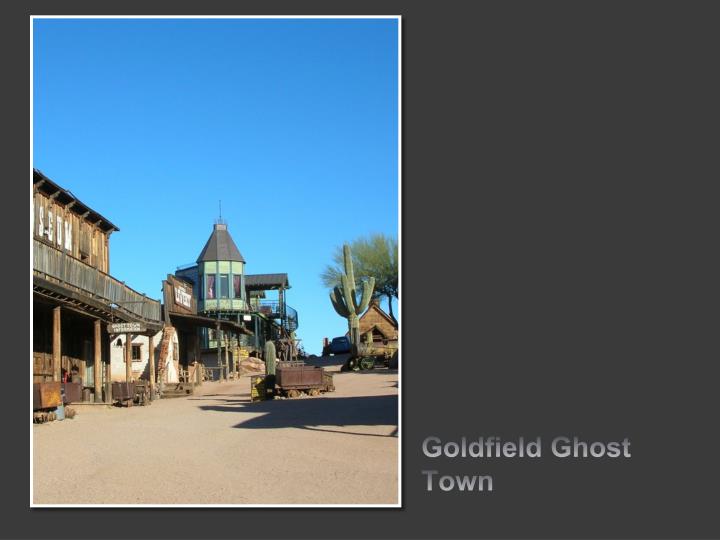The image depicts the revitalized Goldfield Ghost Town, bathed in bright sunlight under a vibrant blue sky. Central to the scene are several buildings that evoke the late 19th to early 20th-century American Wild West style. Dominating the left side is a weather-beaten, two-story wooden structure with a gray balcony and round supporting poles. Adjacent to it is a historically reminiscent green building with a porch held up by pillars. The dirt street in front of these structures is a light brown, casting shadows from the intense sunlight above.

A significant feature in the image is a towering cactus to the right, its main arm reaching approximately 20 feet into the sky, accompanied by multiple smaller arms. A tree with noticeable green leaves also graces the background. Adding to the historic ambiance, a rusted metal cart with wheels is partially buried in the dirt, casting a distinct shadow.

The photograph is framed with a black border, within which "Goldfield Ghost Town" is inscribed in gray letters at the bottom. This detailed portrayal emphasizes the ghost town’s faded yet enduring charm, contrasting against the clear, revitalizing summer day.